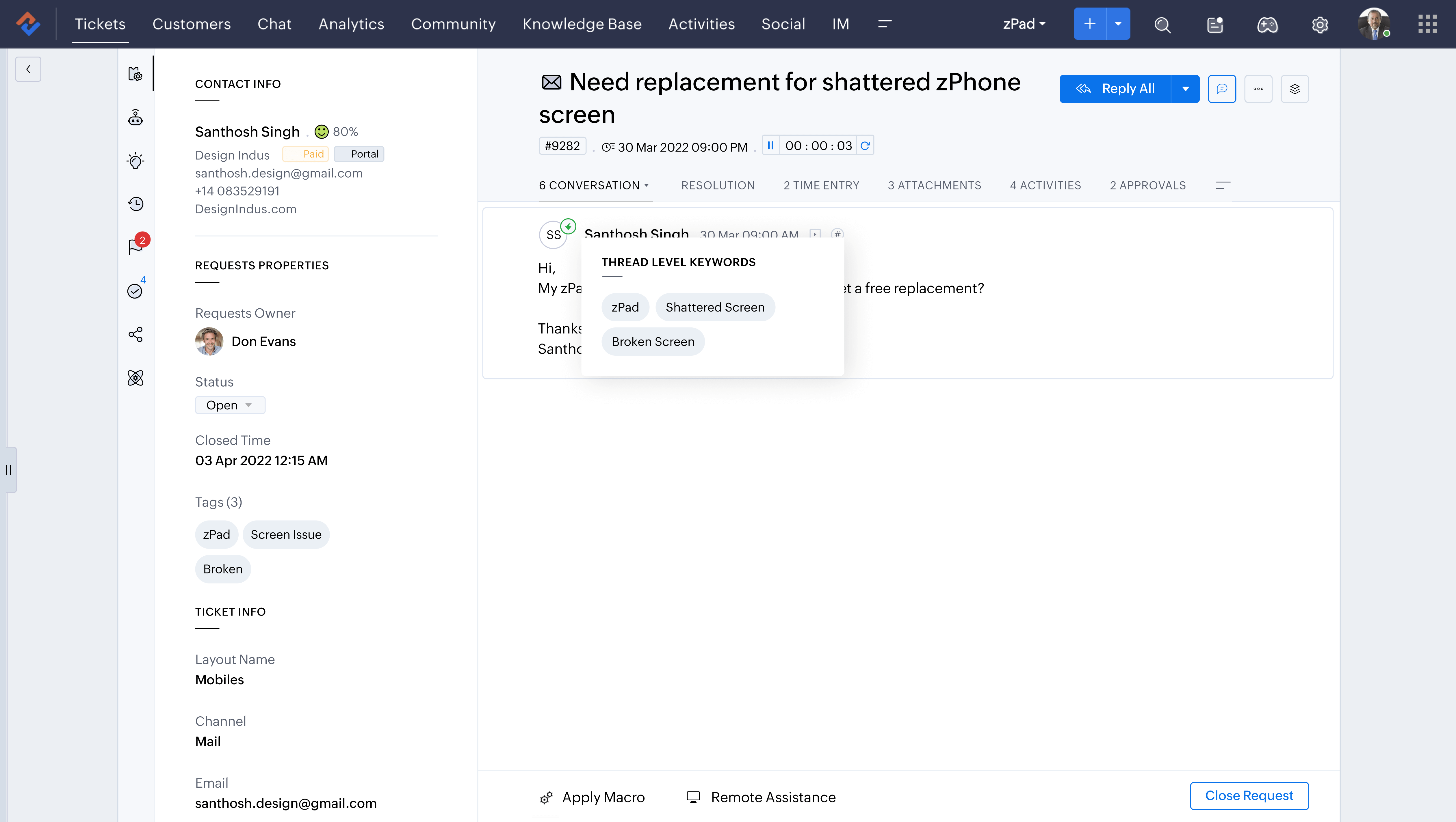This image depicts the user interface of a web application. At the top of the window, there is a black menu bar that spans the entire width of the screen. On the left side of this menu bar, there is a logo resembling a square formed by an inverted "L" and a "J." 

The menu bar includes several menu options labeled as Tickets, Customers, Chat, Analytics, Community, Knowledge Base, Activities, and Social. On the upper right-hand side of the menu bar, a profile picture is visible.

Below the menu bar, the main section of the window is divided into distinct areas. On the far left, there is a vertical sidebar with a margin separating it from the edge of the window. This sidebar contains icons representing different functions or sections of the application. 

To the right of the icon-based sidebar, there is a vertical pane displaying contact information, which includes a person’s name and additional details. This section also highlights the contact’s status or latest activity, indicated by terms like "close time."